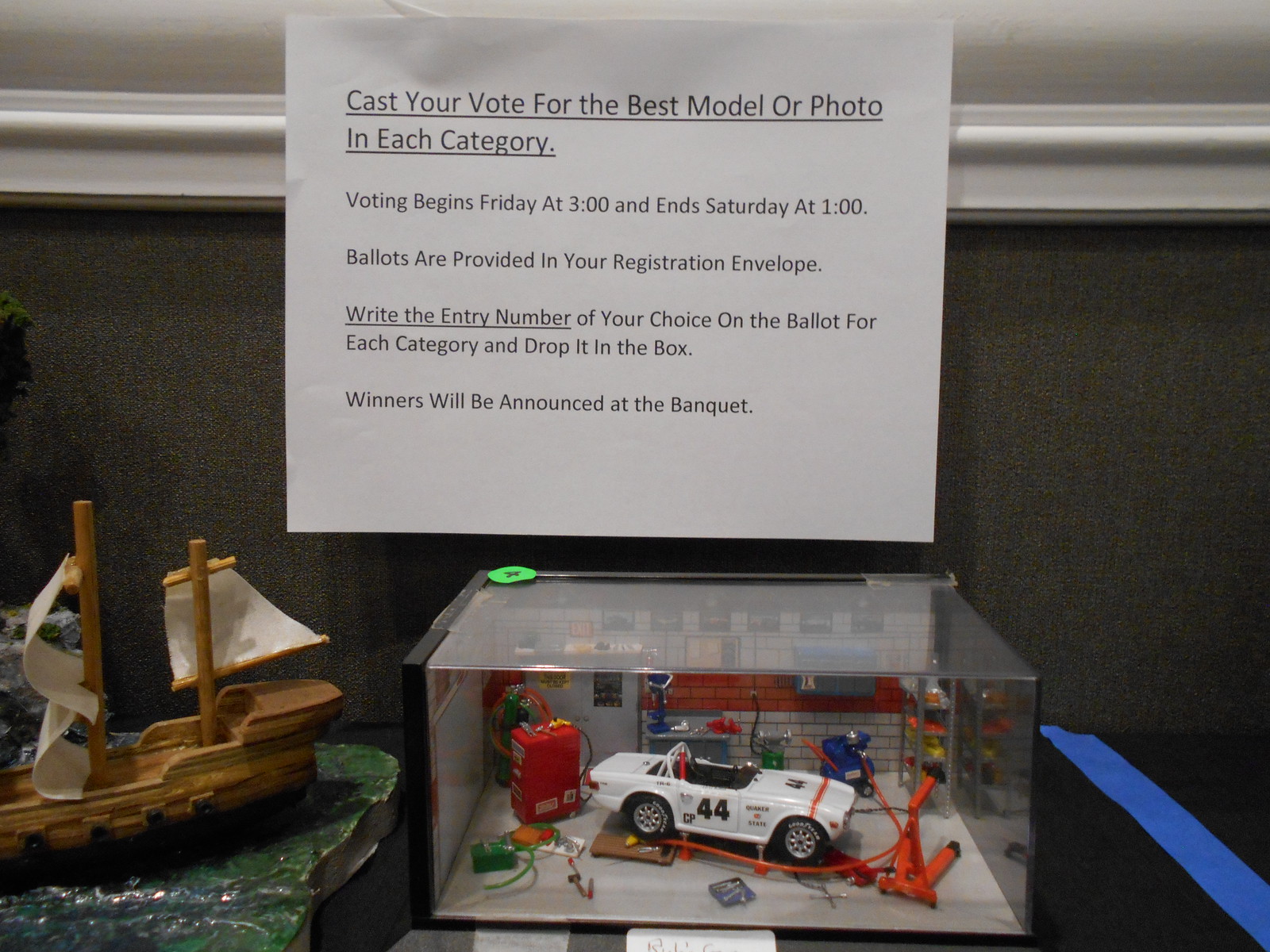In an exhibition room adorned with gray carpeting and a chair railing, a white sheet of paper with black text is prominently displayed, instructing visitors to "Cast your vote for the best model or photo in each category. Voting begins Friday at 3 o'clock and ends Saturday at 1 o'clock. Ballots are provided in your registration envelope. Write the entry number of your choice on the ballot for each category and drop it in the box. Winners will be announced at the banquet." Below this notice, two intricately detailed models stand out. On the right, encased in glass, is a white model car meticulously presented as if in a mechanic shop, complete with tiny repair parts, highlighting its complexity. Adjacent to it, on the left, is a wooden boat model with white sails and two flags, exuding a simple yet elegant design. The entire setup is meticulously arranged, capturing the essence of the displayed models in the competition.